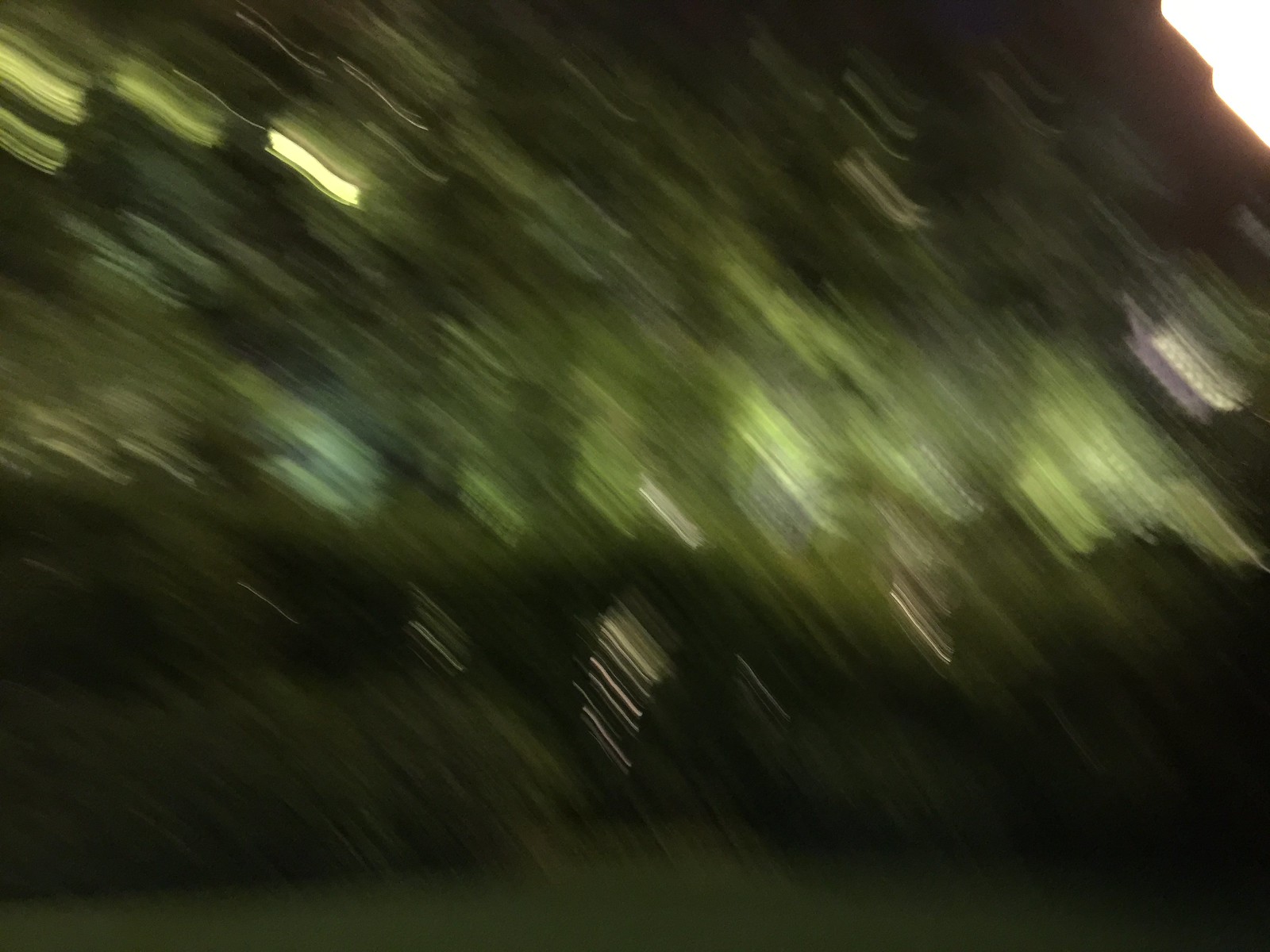The image is a blurry snapshot, likely taken mid-fall in a forest setting. The scene is dominated by a chaotic mix of various shades of green, suggesting grass, bushes, and trees, interspersed with spots of light and darker areas. In the top right corner, a glaring flash of white hints at a camera flash, possibly obscured by a finger. The bottom right corner features a prominent black stripe. The blurry patterns streak diagonally from the top left to the bottom right, reinforcing the impression of hasty movement. The top part of the image might depict trees or a sky softly lit, while the lower section is a blend of medium and darker greens, suggesting dense vegetation. Overall, the photo conveys the disorienting motion of someone falling and snapping a picture in the forest.